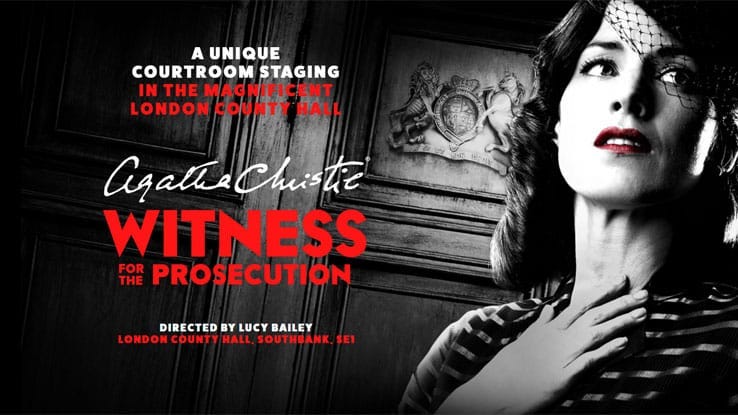In this striking black and white image, which evokes the classic noir style of the 1920s, a woman stands in front of the ornate wooden doors of a courthouse adorned with a royal emblem featuring a lion and a horse crowned over the earth. This is an advertisement for an upcoming theatrical production. The woman, depicted in grayscale except for her bold red lips, wears a black hat with a net covering the right half of her face and holds her right hand to her throat, giving her a distressed appearance.

To the left side of the poster, detailed text announces the event: at the top in white, all capital letters, it reads "A UNIQUE COURTROOM STAGING," followed in red by "IN THE MAGNIFICENT LONDON COUNTY HALL." Below a small space, in elegant cursive white script, it says "Agatha Christie." The title, in larger, bold red letters, proclaims "WITNESS FOR THE PROSECUTION." Further down, in smaller white text, it lists "Directed by Lucy Bailey," and in red text, it reiterates the location: "LONDON COUNTY HALL SOUTH BANK SET." This intricately designed poster captures the essence of the upcoming performance while highlighting its prestigious setting and celebrated director.